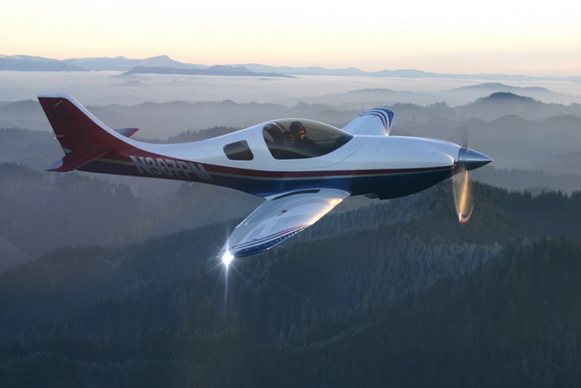This is an image of a small personal airplane in flight, captured from another aircraft. The plane, identifiable by its number N307PM, is predominantly white with a red tail and blue underbelly. It is seen flying over an expansive forested landscape with hilly terrain and a backdrop of distant mountains and fog. The time appears to be around sunrise or sunset, as suggested by the golden hue along the horizon. The airplane's design includes a single engine with a propeller at the front, and it's portrayed flying to the right, visible within the frame. The pilot is discernible through the large cockpit window, though their features remain indistinct. Sunlight is glinting off the right wingtip and reflecting off the plane's propeller, adding a dynamic touch to the scenic vista below.